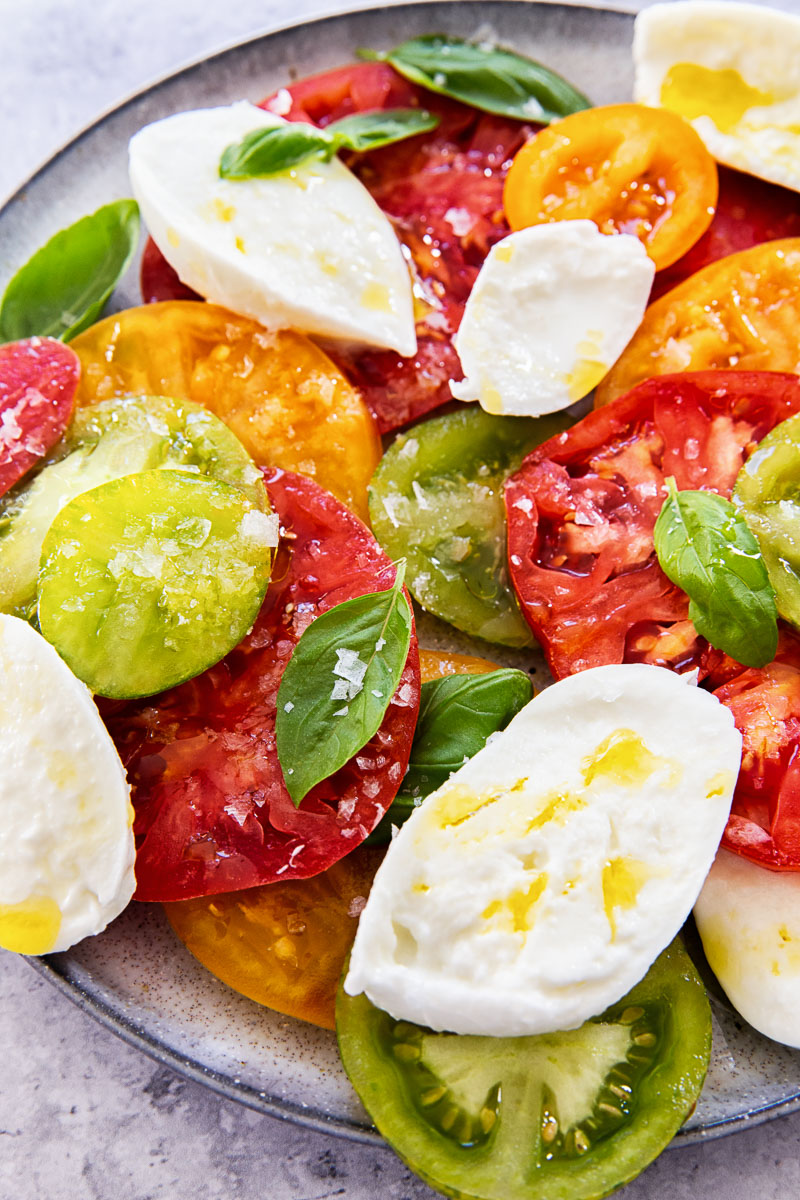This close-up image showcases a vibrant Caprese salad artfully arranged on a white plate with a blue herringbone pattern, placed on a blue marble table. The salad features an array of thinly sliced tomatoes in red, green, and yellowish-orange, complementing the thick, creamy slices of mozzarella cheese. Full basil leaves are interspersed throughout the dish, adding a rich green hue. The salad is generously drizzled with olive oil, making the ingredients glisten, and is sprinkled with coarse sea salt. The presentation, with its professional lighting, evokes an advertisement, emphasizing the fresh and appealing look of the dish. The colors are vivid and inviting, highlighting the juicy tomatoes, fresh basil, and rich mozzarella, all expertly captured to create a visually stunning and appetizing image.